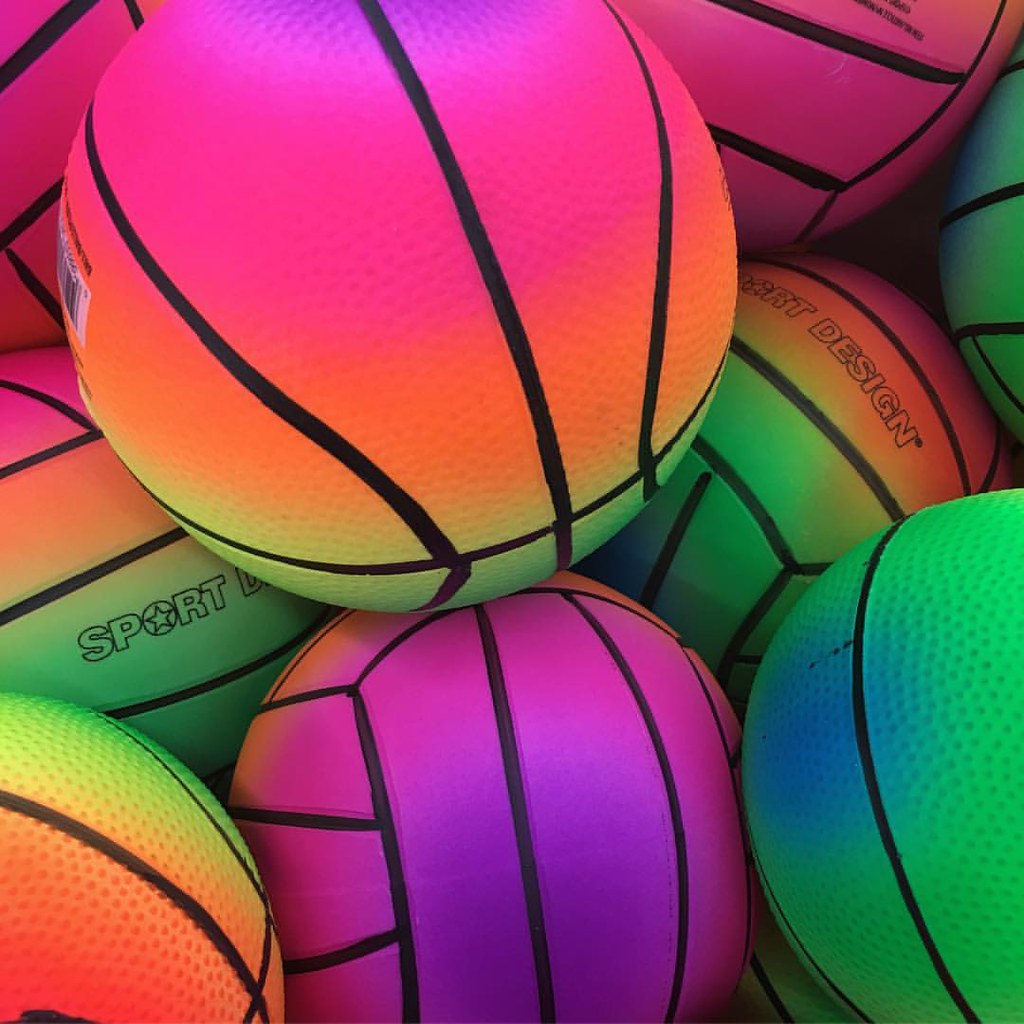This is a close-up photograph of a heap of basketballs and soccer balls, all closely packed together in a container. Each ball features a unique pattern with neon shades of lavender, orange, and green. The design includes sections of these bright colors with black lines separating them, and every ball is stamped with the logo and name of the manufacturer, "Sport Design," in black capital letters. The logo itself consists of a circle with a star inside. Some balls predominantly show purple mixed with orange and pink, while others highlight green and orange layers. The image is so detailed that you can even see the rubber texture and dots on the balls.